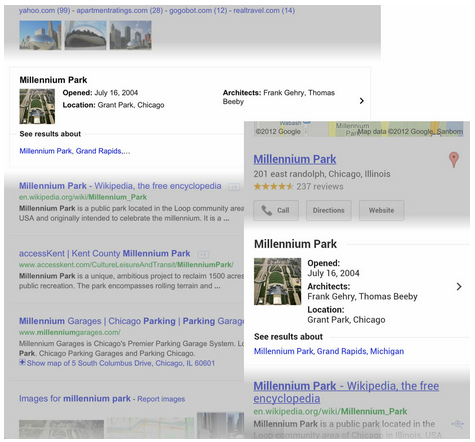The image displays a search results page for "Millennium Park," with two overlapping sections where the smaller one is positioned partially over the larger section. 

**Primary Screenshot:**
- **Main Details (Upper Left):**
  - A small thumbnail image of Millennium Park.
  - Summary information that includes:
    - **Date Opened:** July 16, 2004
    - **Location:** Grant Park, Chicago
  - **Architects:** Features the names of two architects involved with the project.

- **Main Search Results (Center Right):**
  - **Prompt for a Related Search:** "See results about Millennium Park Grand Rapids."
  - **Search Results Listing:**
    - **First Result:**
      - **Title:** "Millennium Park, Wikipedia, the free encyclopedia"
      - **URL:** Displayed in green.
      - **Snippet:** A brief introductory text about Millennium Park.
    - **Second Result:**
      - **Title:** "Access Kent, Kent County Millennium Park"
      - **URL:** Displayed in green.
      - **Snippet:** A brief introductory text about the park in Kent County.
    - **Third Result:**
      - **Title:** "Millennium Garages, Chicago parking, parking garages"
      - **URL:** Displayed in green.
      - **Snippet:** A brief introductory text about parking garages near Millennium Park, Chicago.
 
  - **Additional Media:**
    - **Images for Millennium Park:** Three grayed-out images located at the bottom, only the very tops of which are visible.

**Overlapping Smaller Rectangle (Top Layer):**
- **Header (Blue Text):** "Millennium Park"
- **Information Below:**
  - **Address** and **Reviews:** 5-star rating is visible along with three actionable buttons: "Call," "Directions," and "Website."
- **White Box Content:**
  - **Details:**
    - **Name:** Millennium Park
    - **Opened:**
    - **Architects:**
    - **Location:**
  - **Prompt:** "See results about Millennium Park, Grand Rapids, Michigan"

This overlay mimics the larger section in appearance and content, serving to provide immediate, clickable details about Millennium Park.